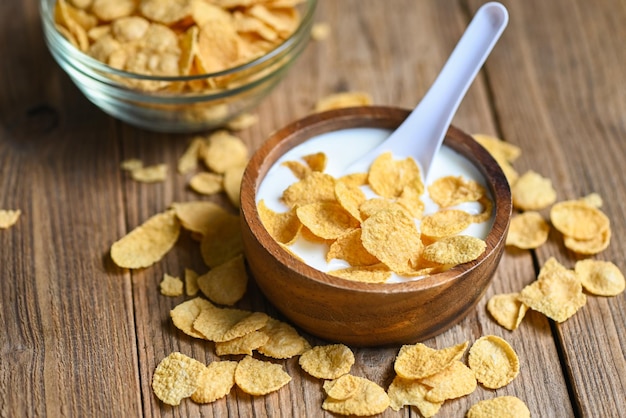In this color photograph with a landscape orientation, the central focus is a small, rounded, brown wooden bowl filled with white milk and golden tan cornflakes. The bowl's rich hue contrasts with the lighter-toned wooden table or countertop beneath, which features dark, almost black grain lines. A white plastic spoon is positioned at an angle in the bowl, its handle extending out towards the top right corner of the image, while the spoon's head is submerged in the milk and cornflakes. Scattered around the bowl are additional cornflakes, hinting at a slightly messy pour. To the top left is a partially visible clear glass bowl, also filled with the same light tan cornflakes. The overall setting presents a clean yet realistic depiction of a common breakfast scene, enhanced by the simplicity of its composition and the quality of the food photography style.